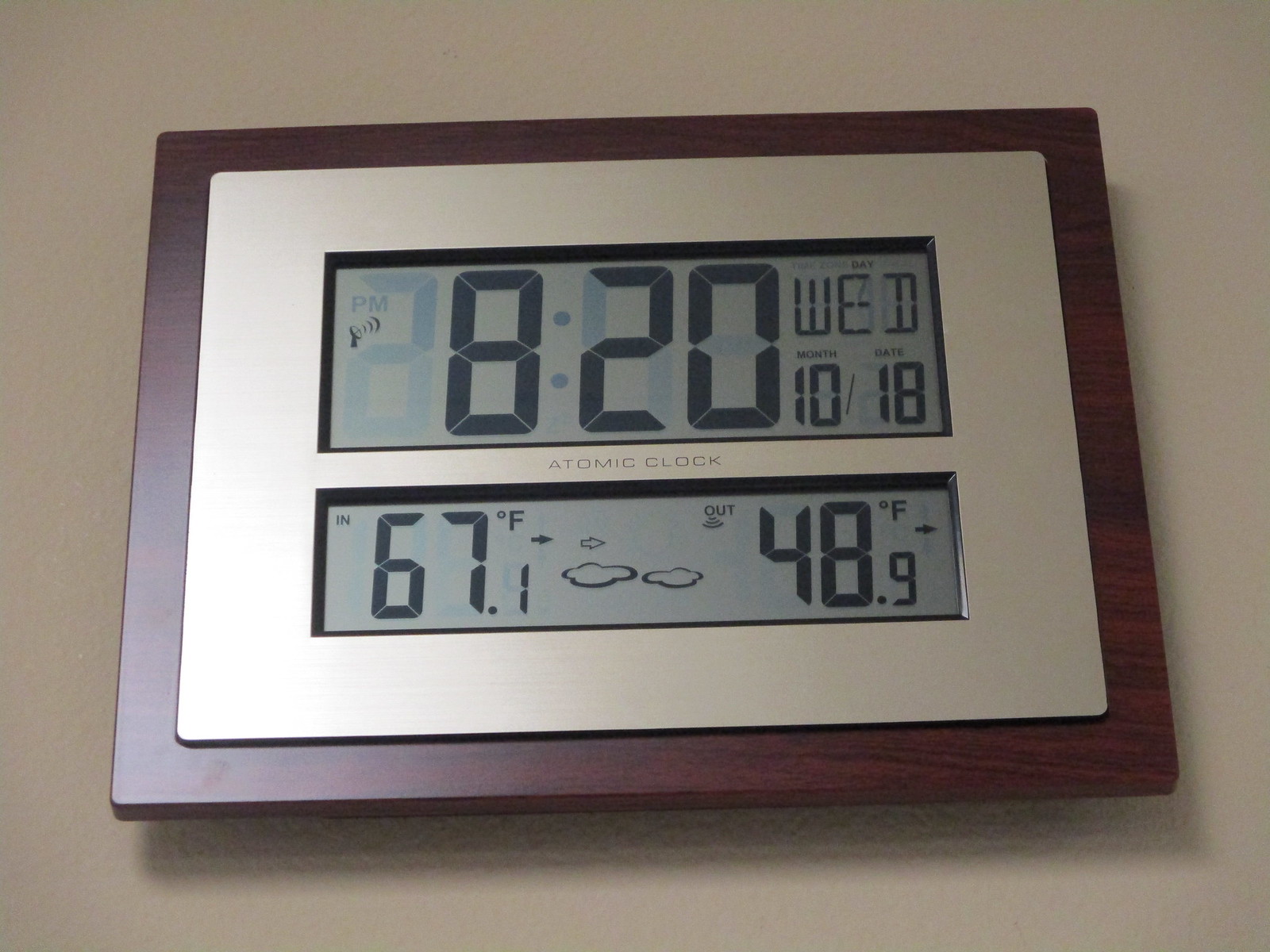This image showcases a unique digital atomic clock mounted on a taupe-colored wall. The clock features a rectangular wooden frame with a silver border inside, enhancing its elegant appearance. The digital display provides comprehensive information: the current time is 8:20 AM, it's Wednesday, October 18th. Additionally, the clock details the indoor temperature at 67.1°F, indicates cloudy weather conditions, and notes that the low temperature from last night was 48.9°F. This multifunctional clock not only tells the time but also keeps track of the date, day of the week, and important temperature data, making it a highly informative and stylish addition to the room.